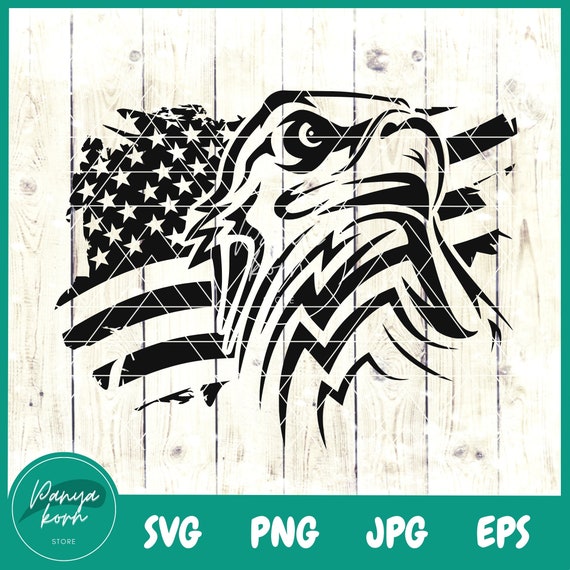This digital store image is a square design framed by a greenish-teal border. The central artwork features a detailed black and white profile of a bald eagle’s head facing right, set against a background that mimics the texture of vertical white wood planks. Behind the eagle, an abstract rendition of the American flag in black and white is partially visible, with a mix of stars and alternating black and white stripes. In the bottom left corner of the border, a white circle contains cursive writing that appears to spell "Panya Korr" above the word "store" in regular font. Adjacent to this, in large, white, capitalized, bubbly letters, are the file format labels “SVG PNG JPG EPS.”